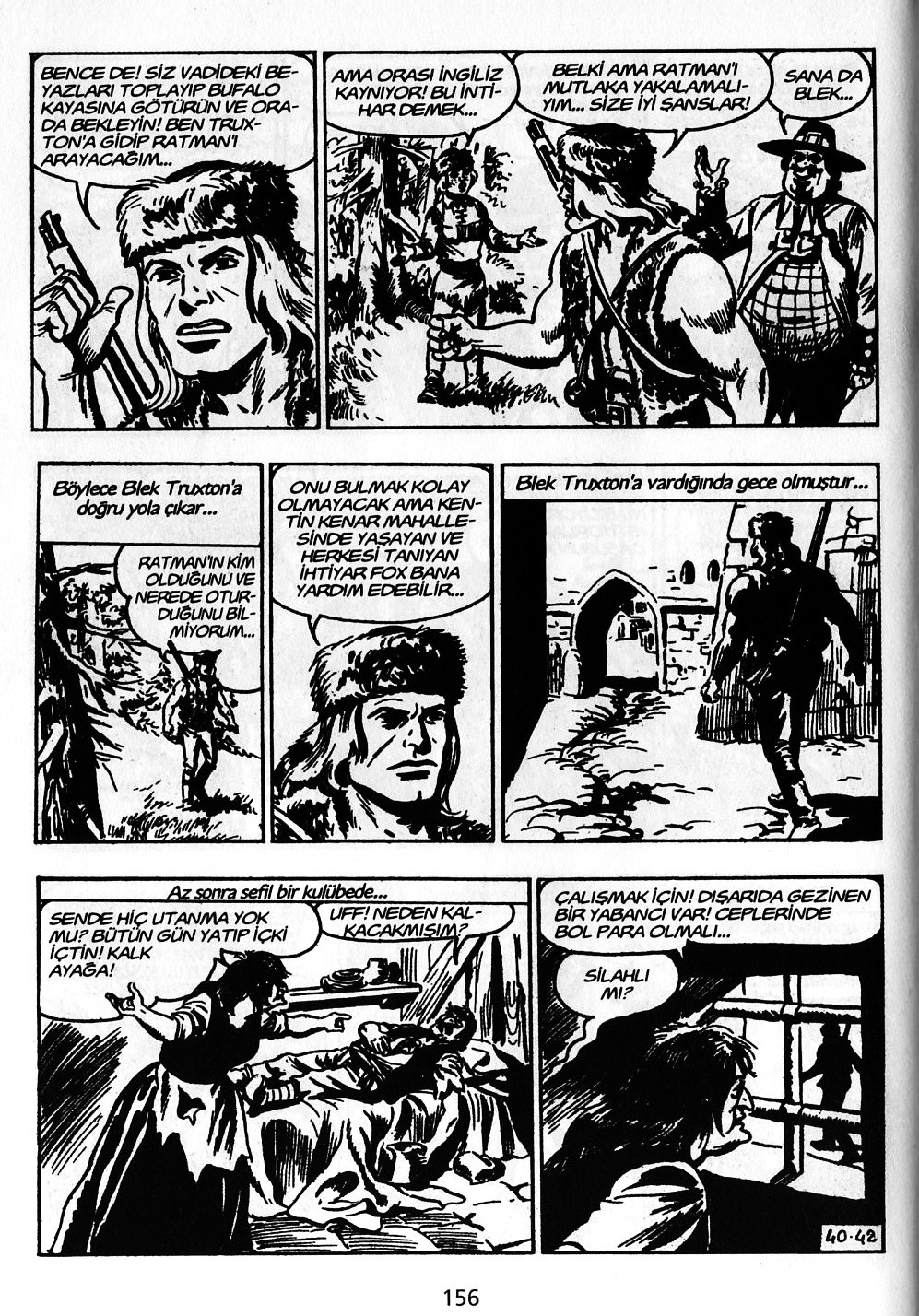This black and white comic book page, marked as page 156, features three rows of panels with text written in Spanish. The narrative revolves around a central character who resembles a mountaineer or frontiersman, donning a fur hat with a raccoon tail, reminiscent of Daniel Boone or Davy Crockett, and carrying a rifle over his shoulder. 

The top row has two panels: the first presents this commando-like character, and in the second panel, he is depicted alongside three men—potentially including an Indian, himself, and another man wearing a hat.

The middle row comprises three panels. The first shows the mountaineer character at a distance. The second is a close-up of his face, and the third portrays him entering a village through a rounded archway.

The bottom row contains two panels: one shows a woman beside a bedridden man, seemingly yelling at him. In the final panel, the woman looks out a window and notices the silhouette of the mountaineer character walking by.